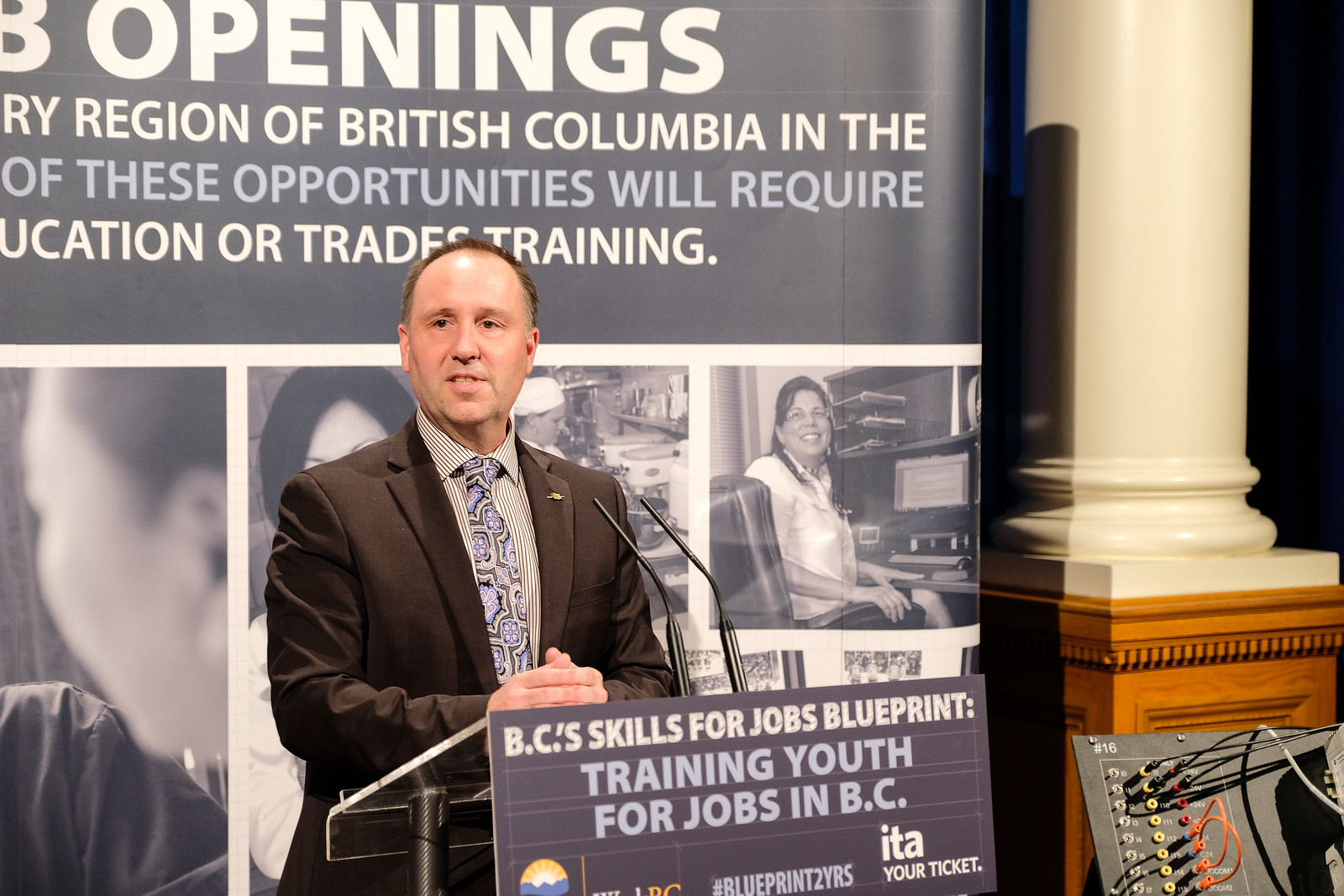A man is delivering a speech at what appears to be a job convention or career-focused event in British Columbia, Canada. He is standing behind a podium, turned slightly to his right, which features a light blue, dark blue, and gray poster stating, "BC's Skills for Jobs Blueprint, training youth for jobs in BC." Additionally, the background includes another poster with partially visible text: "Openings, Region of British Columbia... of these opportunities will require... or trades training." The backdrop also contains black and white images of people working.

The man is wearing a black suit jacket, paired with a striped black and white shirt, and a blue and black tie. He also sports a gold lapel pin and stands with his hands clasped together. Visibly focused, he is intently looking at someone within the room as he speaks. The setting further includes a white Roman-style column with a wooden base to the man's left and an electrical board in the far right corner, likely used for audiovisual support.